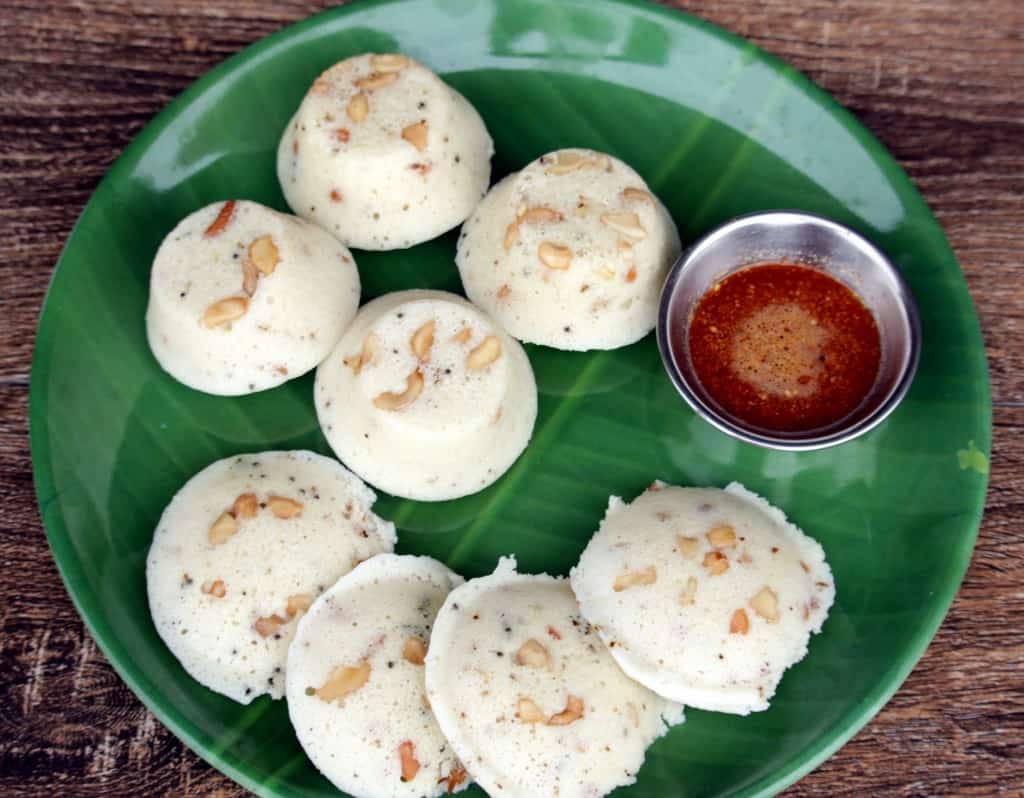The photograph presents a delightful plate of food set on a wooden tabletop, showcasing a meticulously designed dark green ceramic plate with an intricate leaf pattern, complete with visible veins. Arranged around the plate are eight potstickers, which at first glance could be mistaken for sweet cookies or tarts due to their off-white to cream color with black speckles and pieces of nuts or seeds embedded within them. The potstickers have a lightly sprinkled topping, possibly seeds or chopped nuts, adding to their textured appearance. Accompanying the potstickers on the plate is a small, dark silver metal bowl containing a rich, dark red dipping sauce speckled with spices. The entire composition, captured from a top-down perspective, highlights the contrast between the elegant green plate and its delectable contents against the dark brown wood grain of the table, creating a visually appealing and inviting depiction of a savory snack.